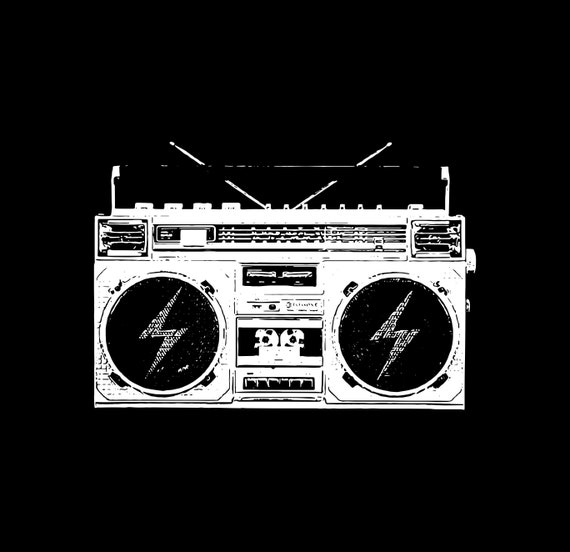This is a detailed black and white graphic image of a 1980s-style boombox set against a black backdrop. The boombox is primarily white with black detailing, prominently featuring two black speaker grills on either side, each adorned with a lightning bolt emblem in the center. Situated in the middle of the boombox is a cassette deck, noticeably empty, flanked below by six black buttons for typical cassette functions such as play, rewind, and record. Above the cassette deck, near the top of the device, are additional buttons and a tuning mechanism, likely for radio frequency adjustments. Two extended metal rabbit ear antennas form a V-shape behind a black handle that spans the full width of the boombox, accentuating its vintage design. On the right-hand side of the device, a prominent knob is present, presumably for changing radio stations. The overall composition captures the quintessential elements of a classic boombox with a modern illustrative twist.